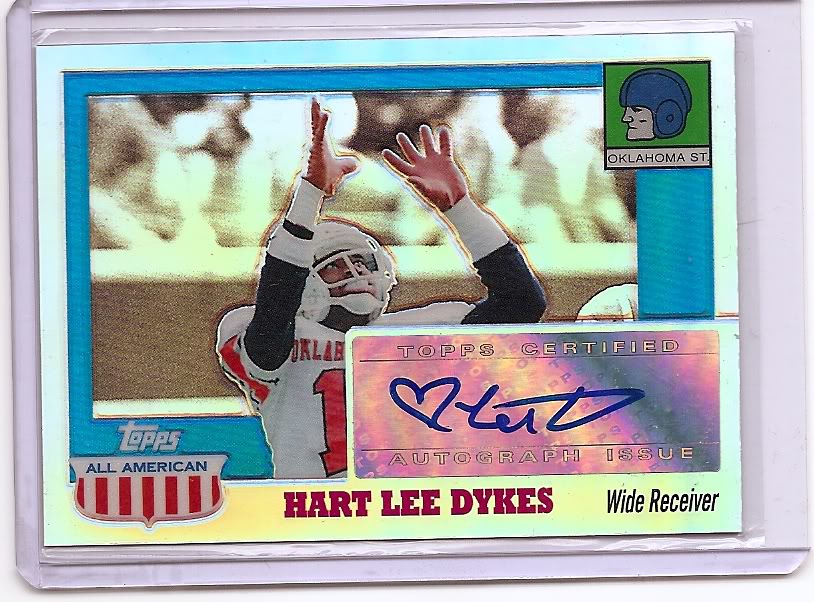This football card features Hartley Dykes, a wide receiver for Oklahoma State, prominently detailed in red text at the bottom of the card. The card, encased in a protective plastic sleeve and holder, is a Tops All-American edition, indicated by the logo with white and red vertical stripes located at the bottom left corner. The central image depicts Dykes making an athletic jump to catch a pass, wearing his white Oklahoma State jersey, marked with a red number one, and accessorized with black sleeves, red gloves, and a white helmet. The card is additionally notable for being a Tops Certified Autograph Issue, with Dykes' signature in blue marker partially covering the player’s image on a light purple plaque. The top right corner features an illustration of an old-fashioned leather football helmet and the words "Oklahoma State." The background also shows a blurred crowd, emphasizing the action on the field.